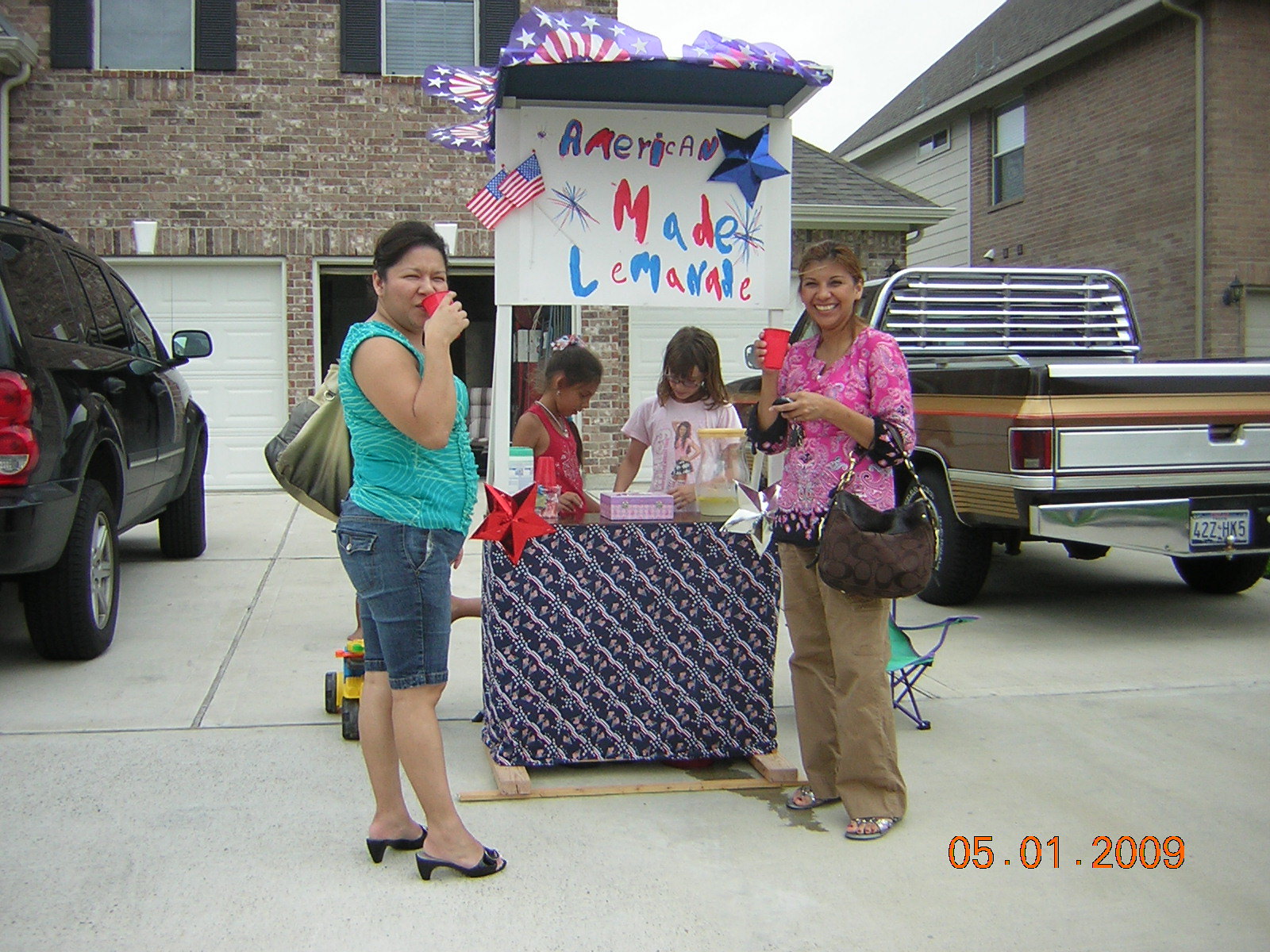This photograph, dated May 1, 2009, vividly captures a charming daytime scene set in the driveway of a brick house with white garage doors. Two young girls, both sporting brown hair and approximately seven years old, are running a wooden lemonade stand adorned with red, white, and blue patriotic decorations and a sign that reads "American-made lemonade." The girl on the left is wearing a red tank top, while the girl on the right is dressed in a light pink shirt and glasses. A small pink change box sits on the front of the stand, which is covered in a blue fabric with red and silver stars.

Flanking the lemonade stand are two women, likely customers, smiling for the camera. The woman on the left is dressed in a teal cut-off shirt, denim capri shorts, and black high heels, holding a red Solo cup in her right hand and a purse on her left arm. The woman on the right wears a pink patterned shirt, tan cargo pants, and a brown coach purse. She also has keys in her left hand and a cup of lemonade in her right.

In the background, you can see a black SUV parked in the driveway and another vehicle, a vintage brown 1970s-style truck, as well as a glimpse of a nearby apartment complex. The scene is sunlit, suggesting a pleasant and warm afternoon perfect for selling lemonade.